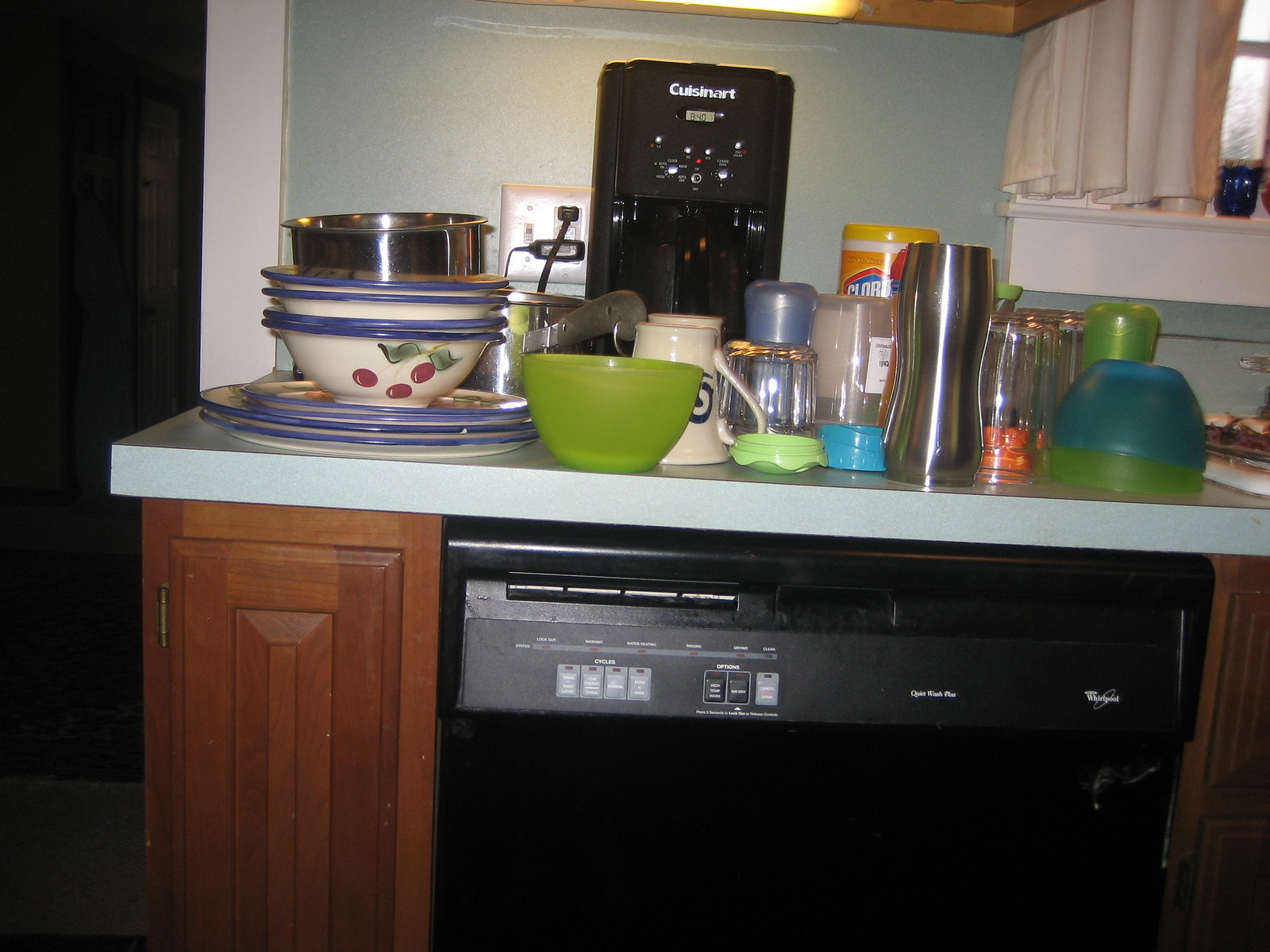This color snapshot captures a slightly messy yet tidy kitchen countertop, photographed at a slight tilt of approximately 5 degrees off horizontal. The light gray countertop is accompanied by wood cabinets below, and prominently features a large double-wide Whirlpool dishwasher. The countertop appears crowded but organized, filled with various clean items. 

On the surface, there are multiple green and blue bowls, some placed upside down, with one green bowl positioned right side up. Among the items is a container that likely holds sugar, a curvaceous metal cup reminiscent of those used for milkshakes, and a bottle of Clorox wipes. Additionally, a black Cuisinart appliance sits on the counter, next to what seems to be a squeeze bottle of syrup. A collection of blue and off-white plates and bowls is also present, with one bowl displaying a cherry motif and blue stripes. A metal mixing bowl adds to the assortment. 

To the right, part of a kitchen window is visible, adorned with an off-white curtain, allowing a glimpse outside. The overall scene provides a snapshot of a busy, actively used kitchen space.